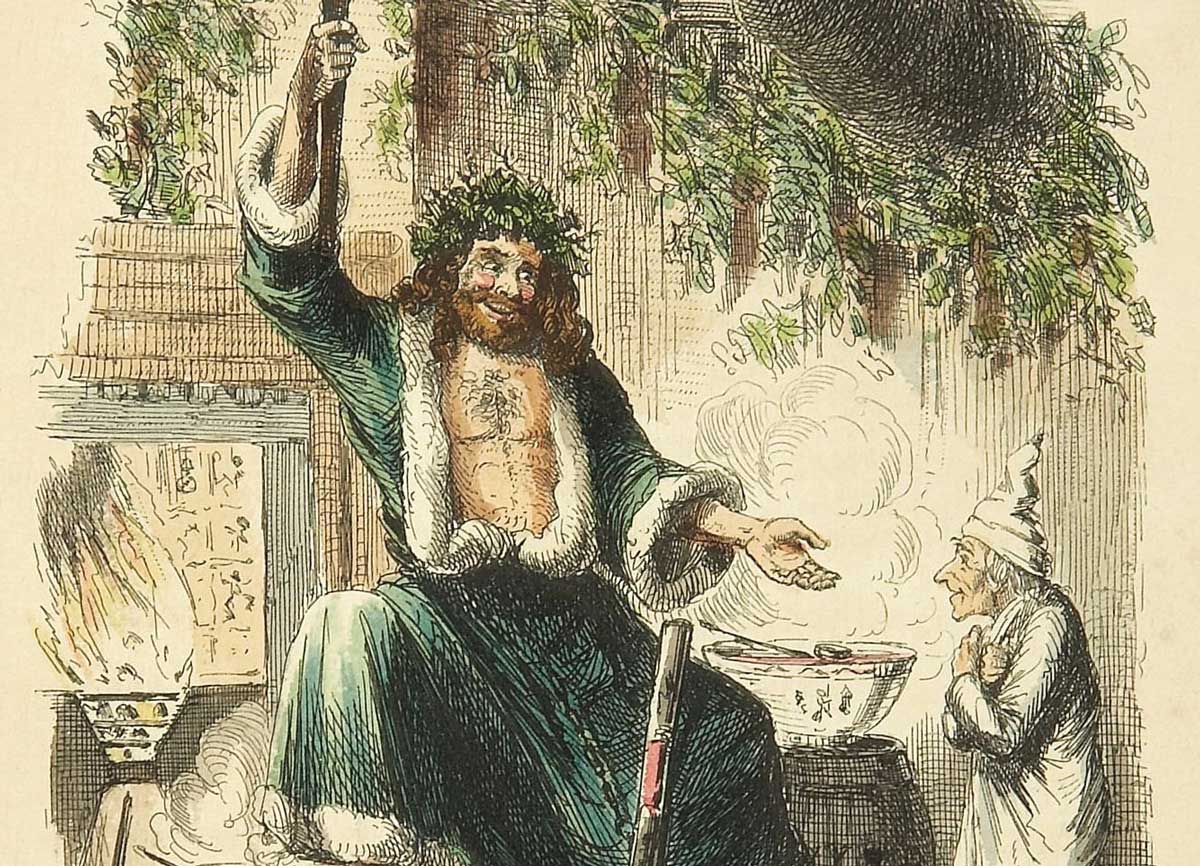The illustration depicts a scene in an older, likely Asian-inspired setting, rendered with a mixture of green, brown, and beige hues on beige paper. Central to the drawing is a large man adorned in a green and white robe, trimmed with fur, exposing his hairy chest. He has long curly hair, a brown beard, and a crown made of foliage, indicating a figure of authority or myth. In his right hand, he holds a staff or torch, while his left hand extends towards an elderly man on his right, dressed in a white robe and a pointy white cap reminiscent of Ebenezer Scrooge. Between them is a bowl emanating steam, possibly soup, sitting atop a barrel. The scene is enriched with additional details such as Asian text on the bowl, a fire in the background, and green shrubbery hanging from above, all contributing to a hand-drawn style reminiscent of historical illustrations. The presence of a building in the backdrop suggests an indoor setting, further emphasizing its antiquated charm.